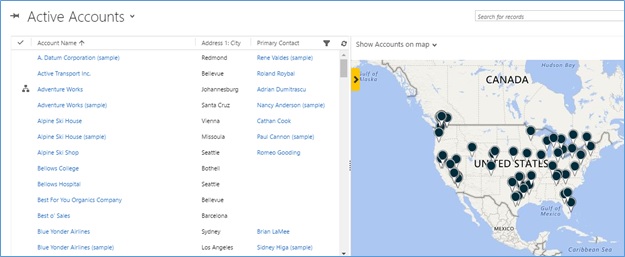The screenshot displays a user interface with an organized and detailed layout. On the upper left, there's a push pin icon pointing to the left, labeled "Active Accounts," accompanied by a dropdown menu. Adjacent to it, on the right, is a search bar that reads "Search for Records."

Below this, on the left side of the screen, a structured chart is showcased. This chart comprises headers titled "Account Name," "Address," "City," and "Primary Contact." Listed under the "Account Name" header, we have a series of entries in alphabetical order, beginning with "Datum Corporation." The list continues with "Active Transport," "Adventure Works," "Adventure Works [unspecified additional detail]," "Aspire" (enumerated thrice), and "Bellows College," along with "Bellows on High."

On the right side of the screen, there is a detailed map spanning Canada, the United States, and Mexico. This map is populated with numerous dots representing active account locations. The United States has a high density of these dots, while Canada has a sparse distribution with dots primarily in the eastern and western regions. Mexico, however, shows no active account dots.

The overall presentation gives a comprehensive view of where the active accounts for this organization are geographically located, while the chart provides detailed specific information on each account.